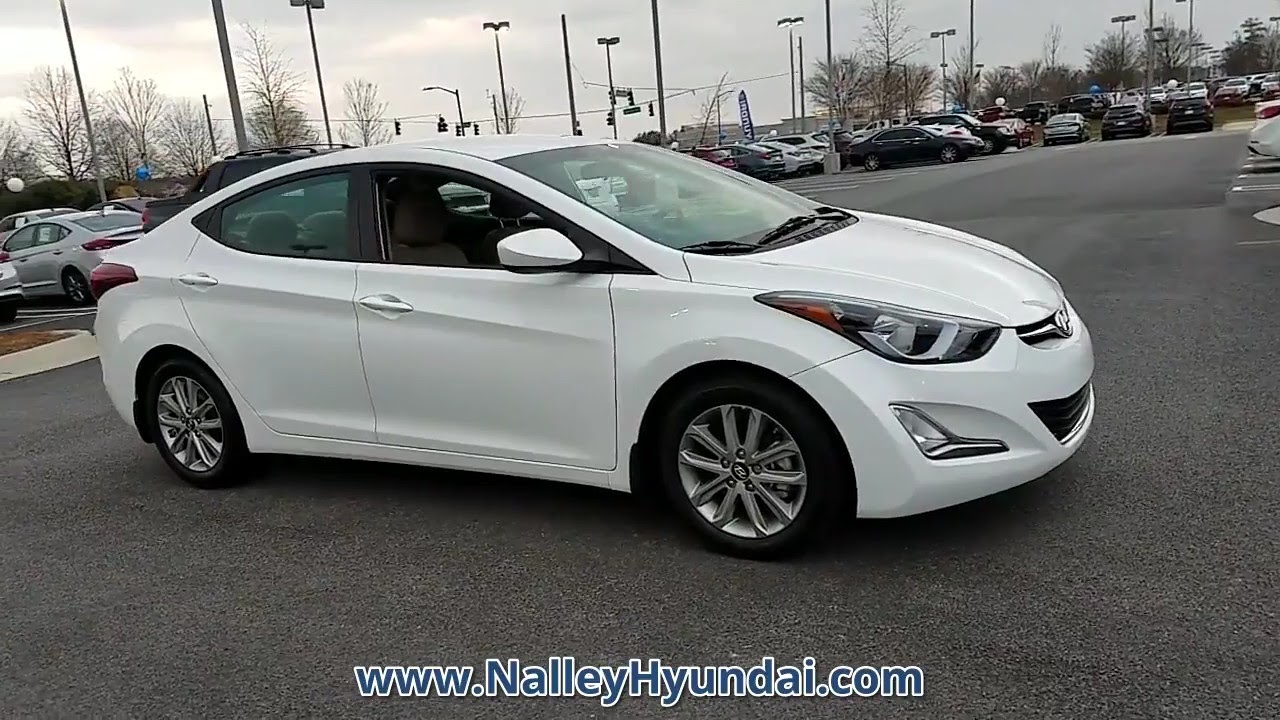This image is of a clean, white Hyundai sedan parked in a large dealership parking lot, signified by the URL nataliehyundai.com written in blue font with a white outline at the bottom of the photograph. The car, likely a new or relatively new 2020s model, features standard wheels and is situated in an organized array of various other vehicles, indicating the dealership setting. The parking lot is filled with numerous cars and is dotted with several light poles. The scene is characterized by a gray, overcast sky, adding a subdued tone to the atmosphere. Off in the distance, other dealership signs and potential balloons can be seen, reinforcing the commercial car lot environment. Additionally, there are delineated parking spaces to the right, likely for customers.